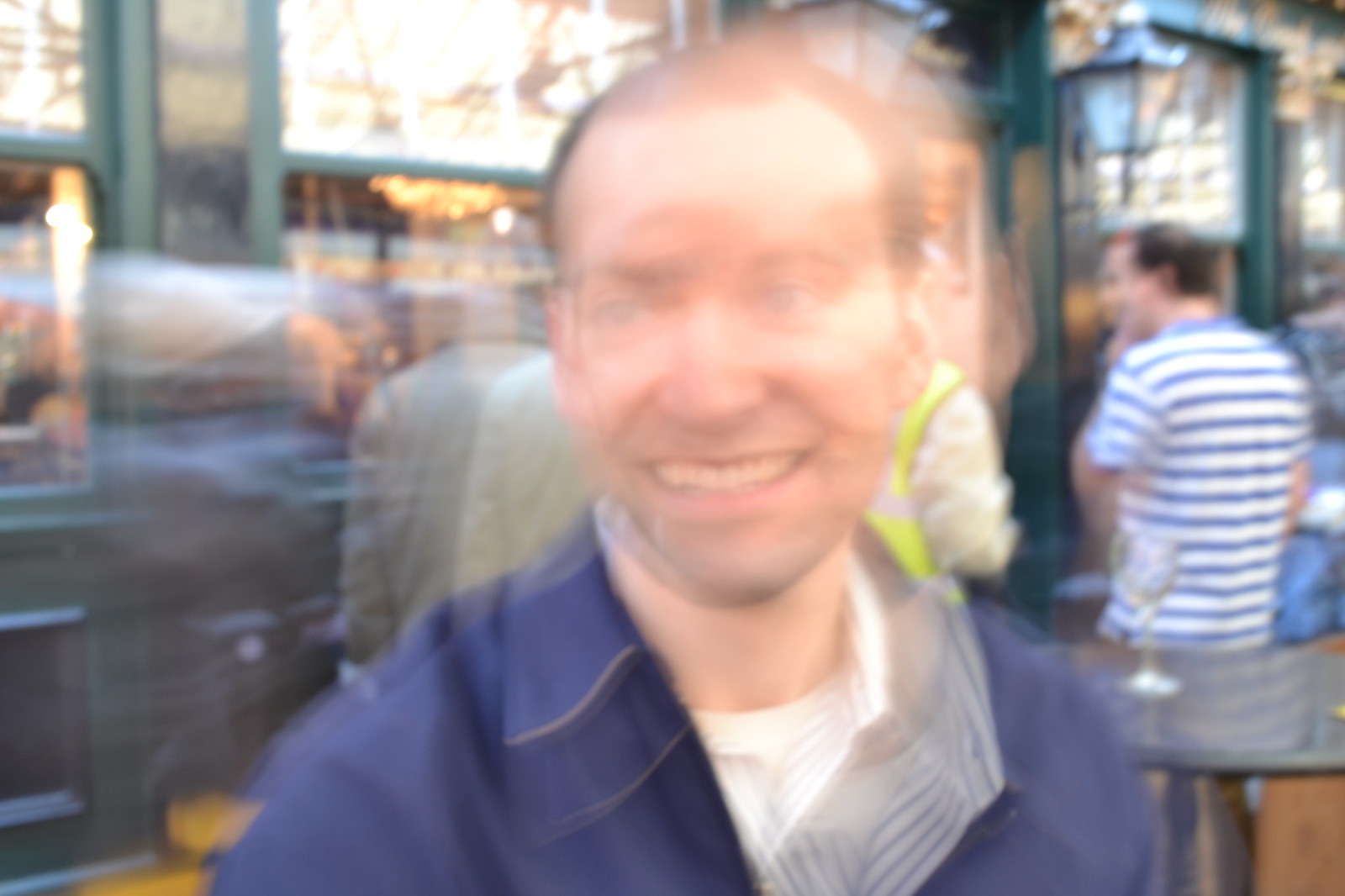In this blurry, out-of-focus photograph, a man stands prominently in the foreground, facing the camera with a warm smile. He has very short, dark hair and appears to have striking blue eyes. He is dressed in a light-colored shirt, layered with a blue jacket. Behind him, a group of individuals are positioned facing away from the camera, creating a sense of depth. One man in the background is distinguishable by his blue and white striped shirt. Another individual, partially visible from the side, is wearing a bright yellow safety vest. The group is standing in front of what appears to be a storefront or a business establishment, adding context to the scene. Although the image lacks sharpness, the subjects and their attire provide enough details to convey a sense of their environment and activities.